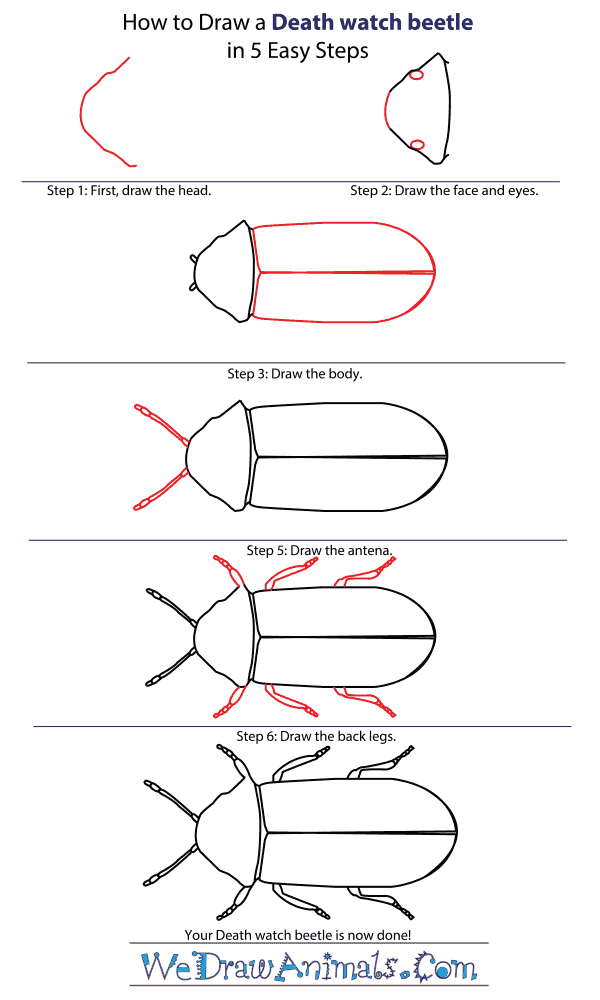This infographic tutorial, titled "How to Draw a Death Watch Beetle in Five Easy Steps" from wedrawanimals.com, features a plain white background with no borders. The title is prominently displayed at the top in bold, black print, with "Death Watch Beetle" slightly larger. The tutorial uses a combination of red and black lines: red to indicate new drawings in each step and black for already completed parts. 

1. **Step One:** It instructs to draw the head, depicted as a rounded shape starting at the top center and curving outward and down. 
2. **Step Two:** This step is about adding the face and eyes to the head, with the eyes drawn in red and connecting lines around reaching black to integrate with the head.
3. **Step Three:** Here, the body is added, described as a long, cylindrical shape divided down the middle.
4. **Step Four:** The antennae are drawn next; two red lines extend from the head.
5. **Step Five:** Finally, the beetle's back legs are added, showing six legs in total.

The last line confirms the completion with "Your death watch beetle is now done," followed by a small blue-accented note of the tutorial's source and website, wedrawanimals.com. Despite some mislabeling in the step order in the narrative, the overall illustrated steps remain clear and sequential.